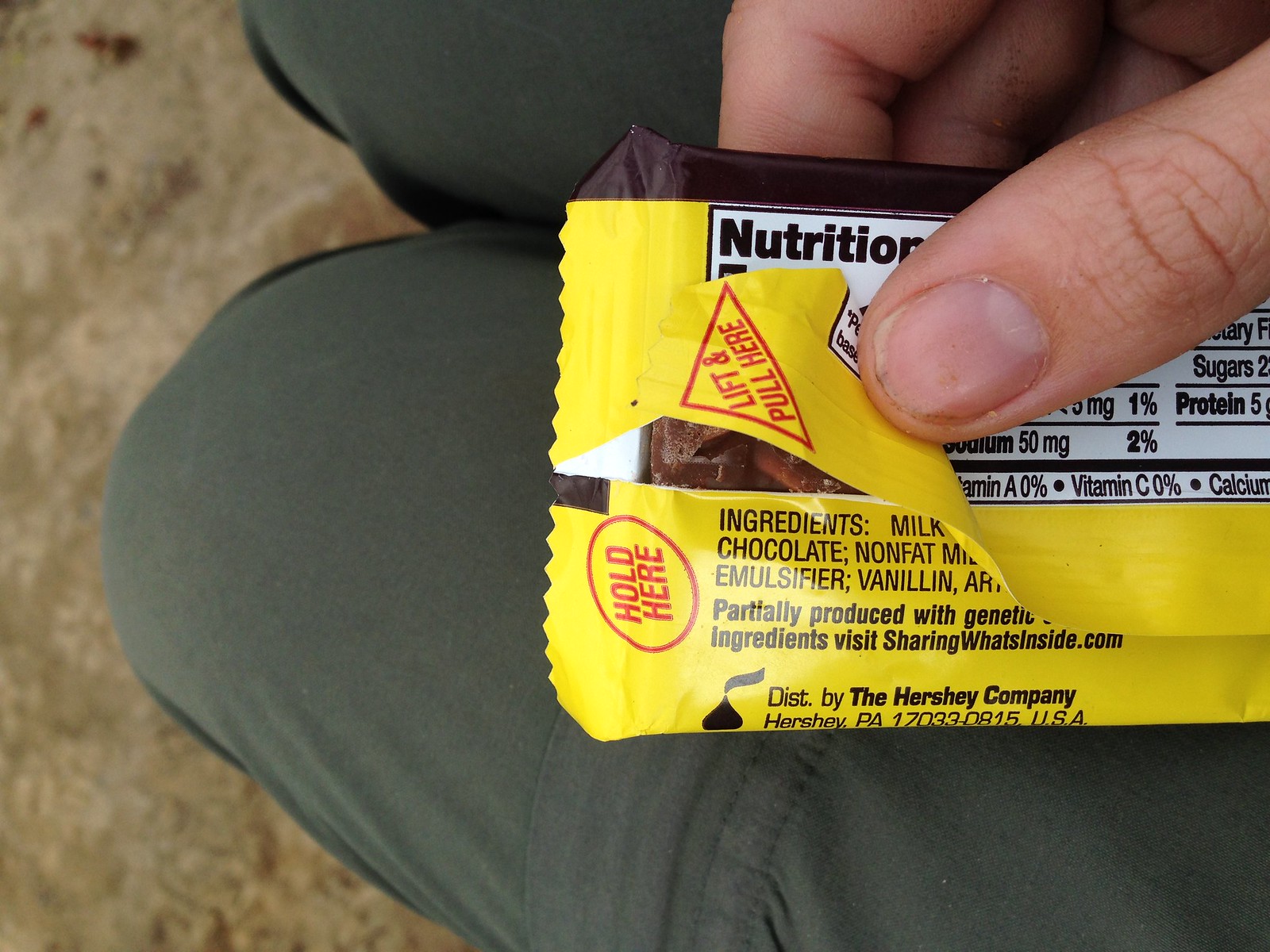In this crystal-clear photograph, a partially opened candy wrapper reveals a piece of dark brown chocolate. A person's thumb and a few fingers are grasping the wrapper, while their gray pant legs indicate they are in a kneeling position on a concrete surface. The candy wrapper is predominantly yellow and features a red circle with the text "Hold Here." Another instruction, "Lift and Pull Here," is visible on the opposite side. Part of the ingredients list can be seen, written in black font, along with a partially visible nutrition facts label. The bottom of the wrapper states, "Distributed by the Hershey Company, Hershey, Pennsylvania," complete with a zip code. Additionally, a chocolate kiss icon is clearly visible, further identifying the brand.